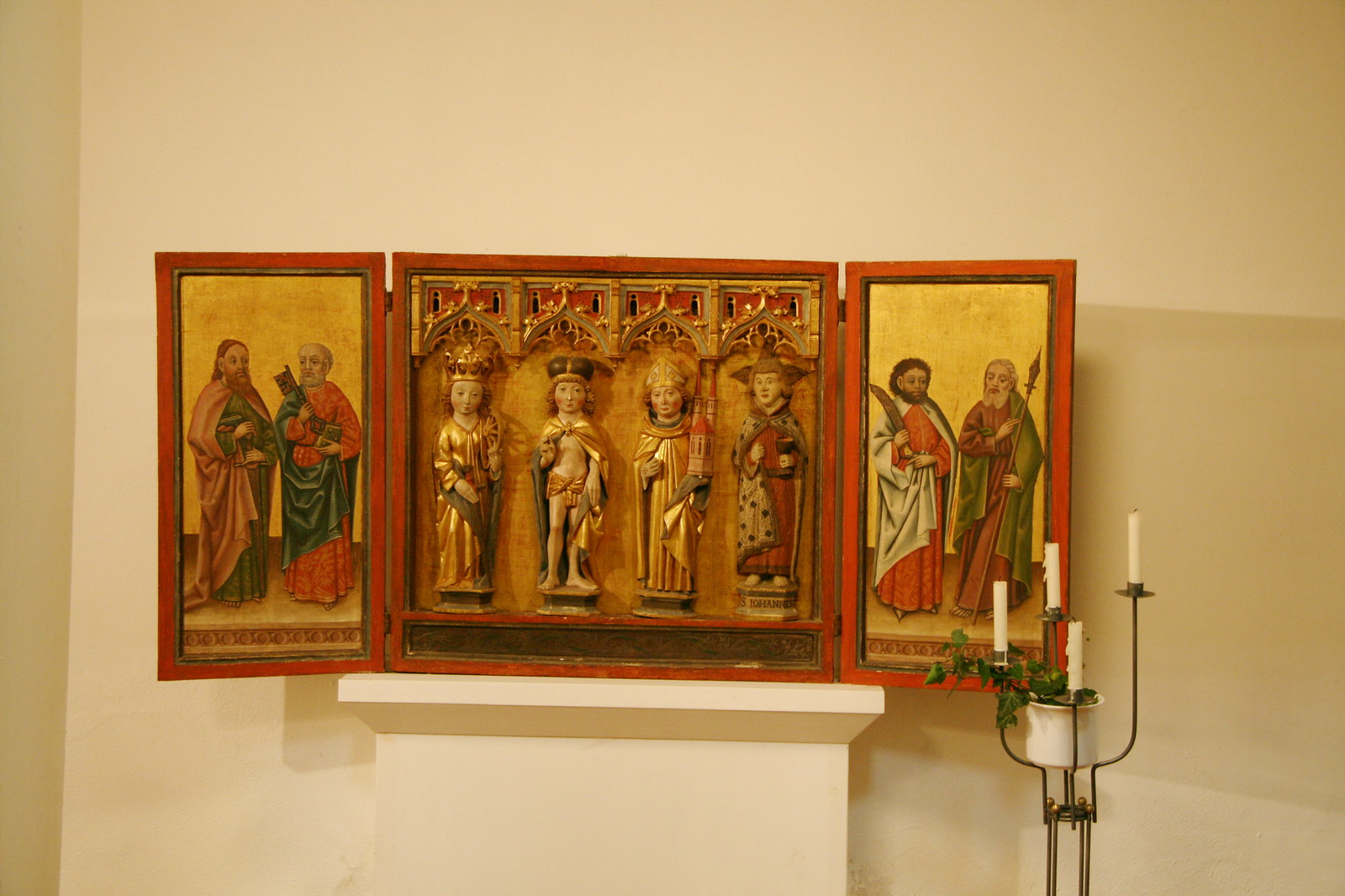This photograph features a detailed arrangement of ancient, religious artwork displayed on a mantle against a white wall. Central to the image is a red wooden fixture with three panels—the middle panel holding four small, raised sculptures of wise men, possibly saints or disciples. The wise men, clad in detailed robes, include one holding an old-fashioned key and another carrying an ink pen feather. Flanking the central panel, each of the two side panels displays a painting of two robed figures, further contributing to the religious theme.

The entire setup is complemented by a black and gold candle holder positioned in the bottom right corner, featuring four lit candles and adorned with green leaves. The scene is framed by the vivid colors of gold, white, brown, and red from the artwork, blending harmoniously with the white backdrop and the warmth of the candles, creating a reverent and serene atmosphere. There is no identifying text or people in the photograph, allowing the intricate details of the religious imagery and the symbolic objects to capture the viewer’s attention fully.